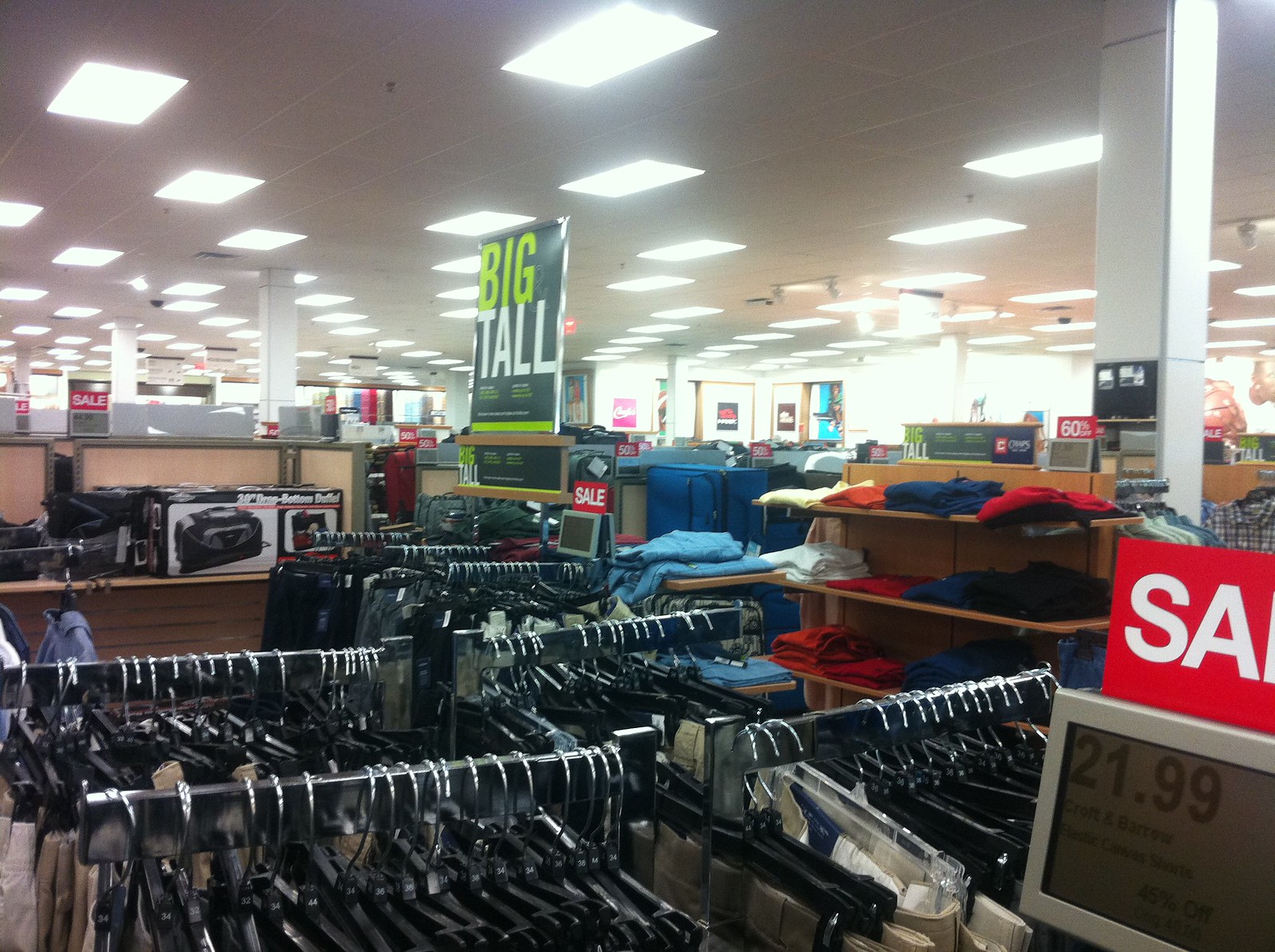The photograph depicts the interior of a department store, specifically focusing on the clothing section. Overhead, the ceiling is adorned with classic rectangular ceiling tiles interspersed with rectangular fluorescent lights. Prominent in the image are multiple racks of clothing; there are two long racks at the bottom of the image flanked by three smaller ones. To the right, shelves—likely made of faux wood—support neatly folded clothes in various colors including red, blue, and white. 

A prominent sale sign, characterized by white lettering on a red background displaying partial letters "S-A", is situated atop a computer monitor. A price tag hanging on one of the clothing racks reads "$21.99", labeling Croft & Barrow elastic canvas shorts with a 45% discount from an original price, which seems to have been roughly $42. Additionally, another sale sign in the background boasts a "60% off" discount, adding to the store's promotional atmosphere. A large banner hangs from the ceiling, indicating the "Big & Tall" section with "BIG" in green capital letters and "TALL" in white capital letters. Scattered throughout the scene are various other sale signs, reinforcing the bustling retail environment typical of department stores, possibly suggesting a place like Kohl's.